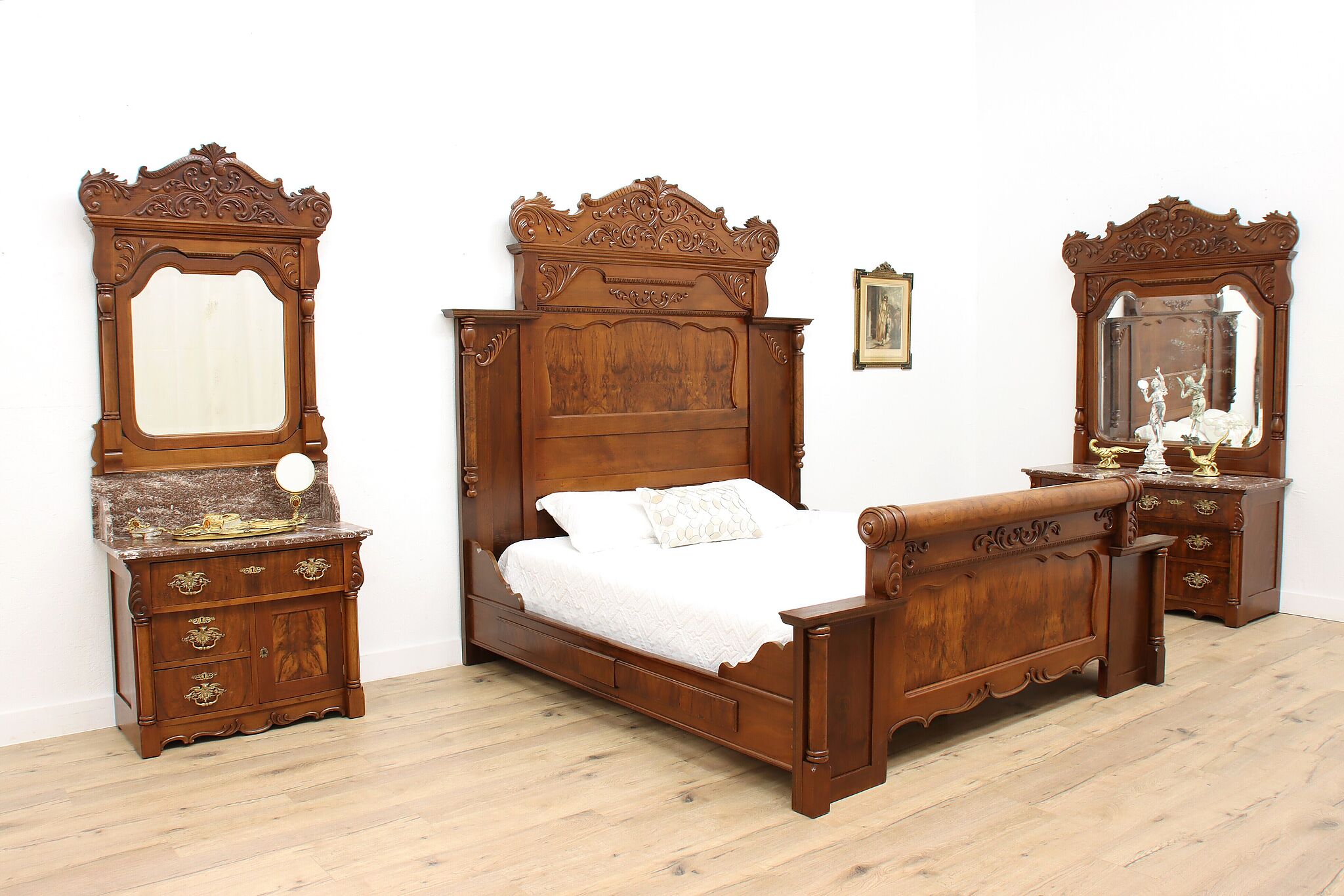The photo captures a meticulously arranged bedroom that features ornate Victorian-style furniture, all crafted from dark brown wood with intricate carvings. In the center of the room is an elaborate bed with a large, ornate headboard and footrest. The bed is adorned with white sheets, two regular white pillows, and a central decorative white pillow with golden details. Flanking the bed are two substantial wooden pieces of furniture, each housing multiple drawers with golden handles. To the left is a vanity featuring a large drawer at the top and three smaller drawers underneath, topped with a mirror that replicates the wood's ornate carvings. On the vanity, there is a light and a golden tray among other objects. On the right side, there is a chest of drawers, again with a large mirror reflecting the bed's headboard. The chest holds a collection of trophies and golden statues. The room's white walls are complemented by light brown wooden flooring, and a framed picture hangs on the wall beside the right side of the bed, encased in an ornate frame matching the rest of the furnishings. The overall atmosphere of the room is clean, well-ordered, and exudes a sense of historical elegance.